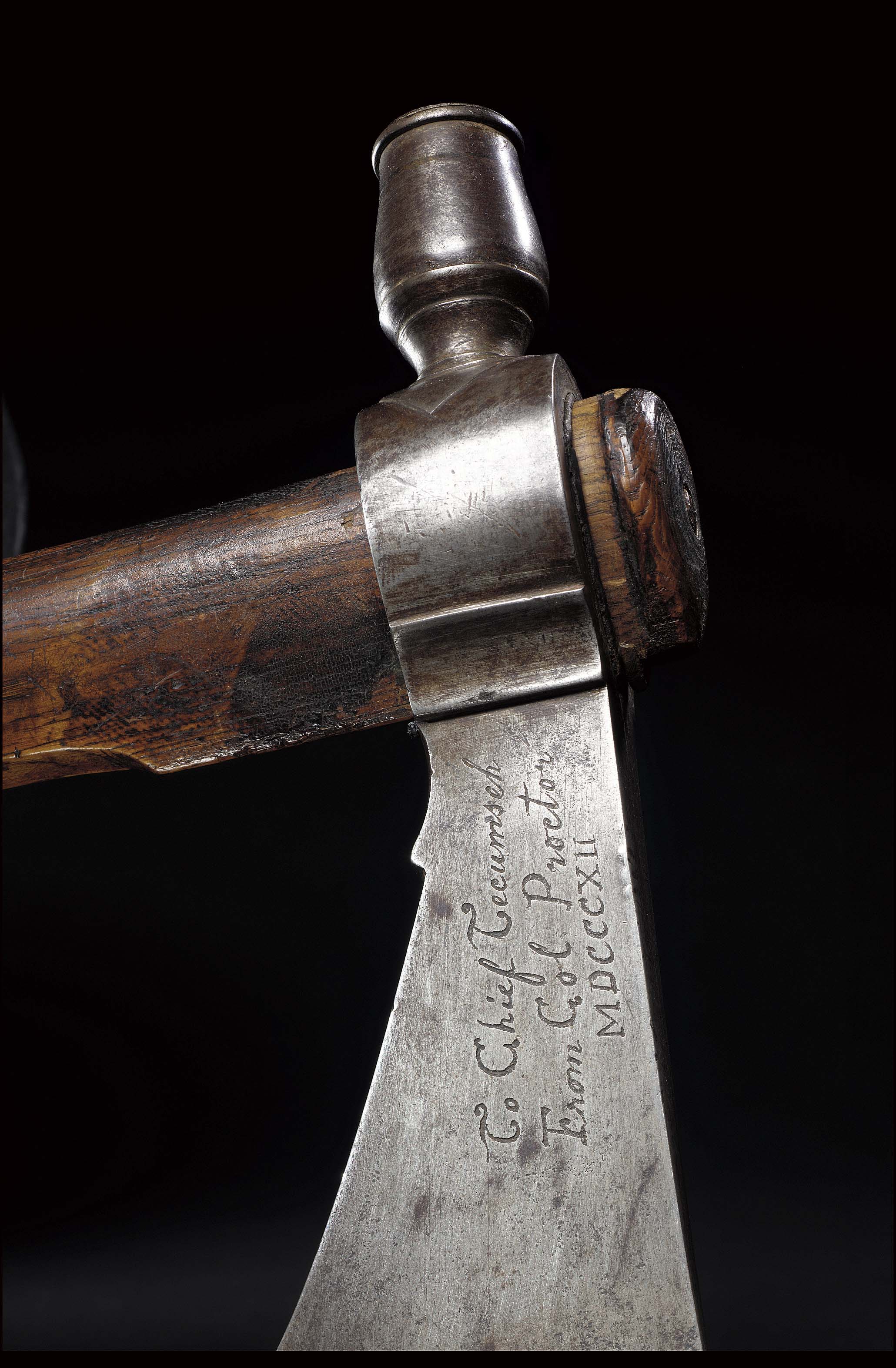The photograph showcases a close-up view of a ceremonial hatchet against a black background. The image emphasizes the aged, silver metallic blade of the hatchet, which takes up the central focus, with only a sliver of the dark brown wooden handle visible. Engraved in cursive on the blade is a dedication to Chief Tecumseh from Colonel Proctor, along with the date inscribed in Roman numerals as "MDCCCXII." The detailed engraving and the historical significance of this gift highlight its cultural importance and link to the heritage of Chief Tecumseh.